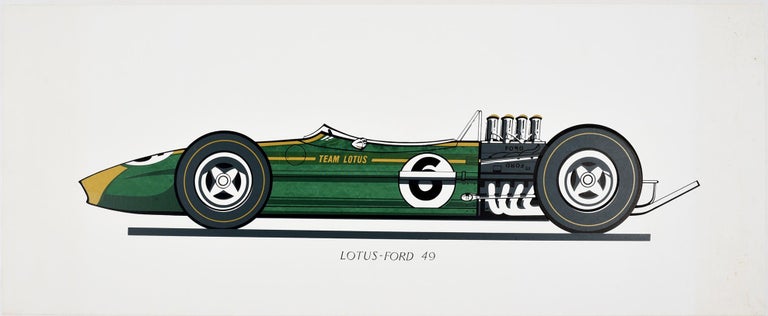This image is a highly detailed, professional drawing of a vintage race car, specifically a Lotus Ford 49, set against a stark white background with no other elements. Dominantly green with vibrant yellow accents, the car features yellow pinstripes and racing stripes along its front. Written in golden letters along the side, "Team Lotus" is prominently displayed, along with a large, black number 6 outlined in white. The car is oriented to the left, showcasing its two oversized black tires which rise above the car's body profile. The depiction emphasizes the car's powerful rear engine, which occupies about 30% of the vehicle's length and includes visible exhaust pipes. Overall, the illustration conveys the sleek, streamlined design and historical significance of this classic race car, likely from around 1949 as suggested by the model name and era-specific details.